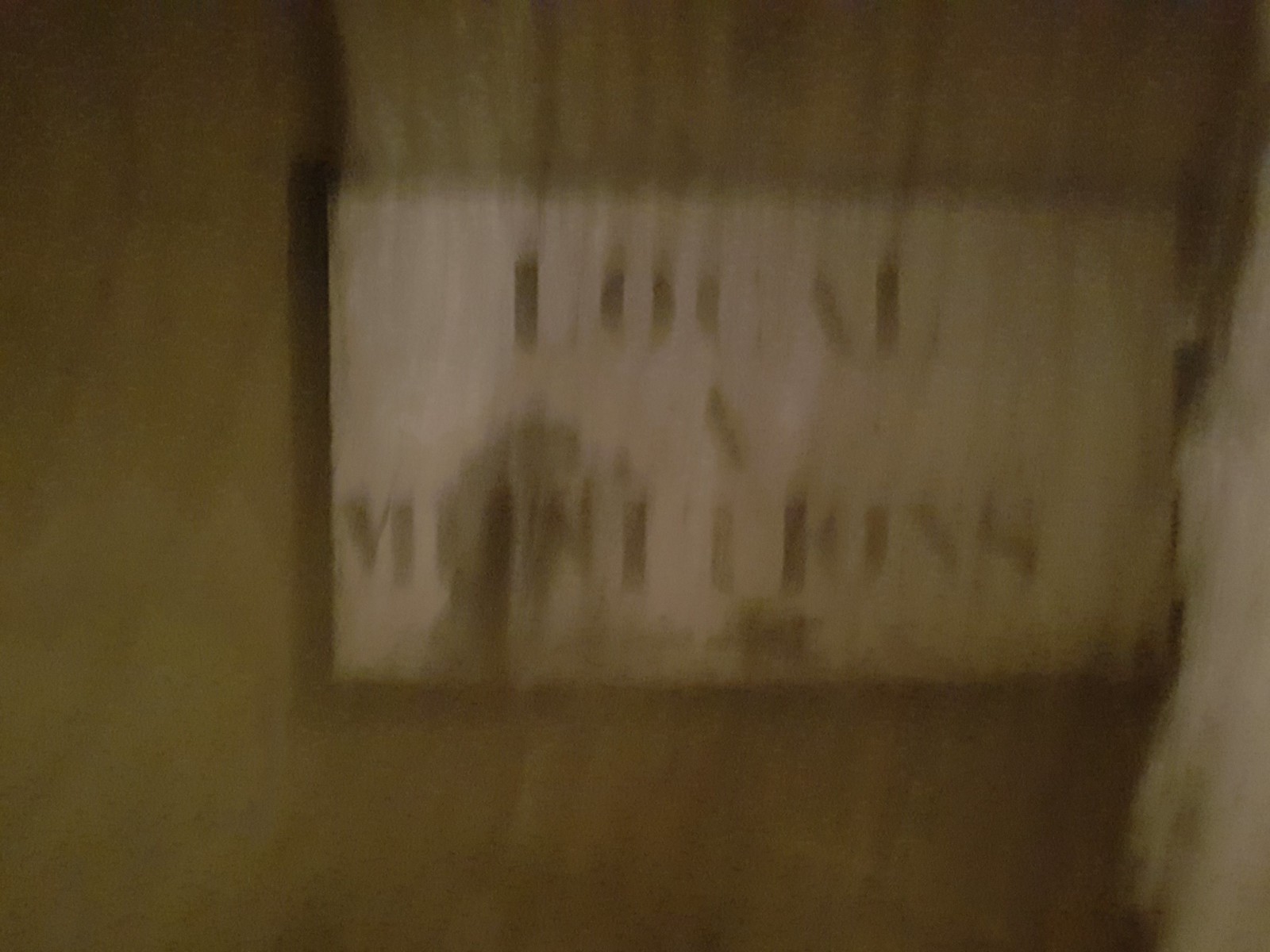The image depicts a very blurry rectangular framed sign attached to a wall, enveloped in shades of light brown, dark brown, and a dull beige color. The sign appears to be a slightly dirty white or cream-tan color with black printed letters. The top line of the text on the sign seems to clearly spell out "LOCAL." However, the subsequent lines are difficult to decipher due to the motion blur and faded print, with the second line appearing to start with an "M" and potentially ending with "I-O-N-S," but the exact text remains illegible. The overall blurriness of the image obscures precise details, rendering the full content of the sign unintelligible.